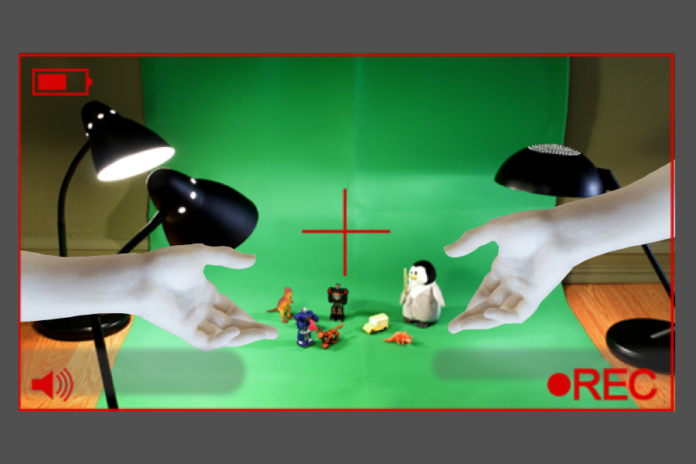The image is a screenshot of a video camera recording a claymation setup. The frame is outlined by a thin red rectangle, indicating the camera’s viewfinder against a gray background. At the top left, there is a red battery symbol showing that the battery is partly used, accompanied by a speaker icon indicating the sound is on. In the bottom right, "REC" and a red recording circle icon are visible. Dominating the center of the image is a green screen backdrop situated on a wooden floor, extending upwards onto a gray wall. A red crosshair marks the center of the screen.

Illuminating the scene are three table lamps: two black cone-shaped lamps to the left and one dome-shaped on the right. The green backdrop is adorned with various small toys and figurines, including a stuffed penguin, two robots, two dinosaurs (one resembling a T-Rex), a box truck, a possibly dog-shaped figure, and a large, cartoonish woman character. Colors of these toys vary, including white, purple, black, and orange, arranged on a wooden desk-like surface. Two light-skinned hands, one from the left and one from the right, are poised as if adjusting the positions of these miniatures.